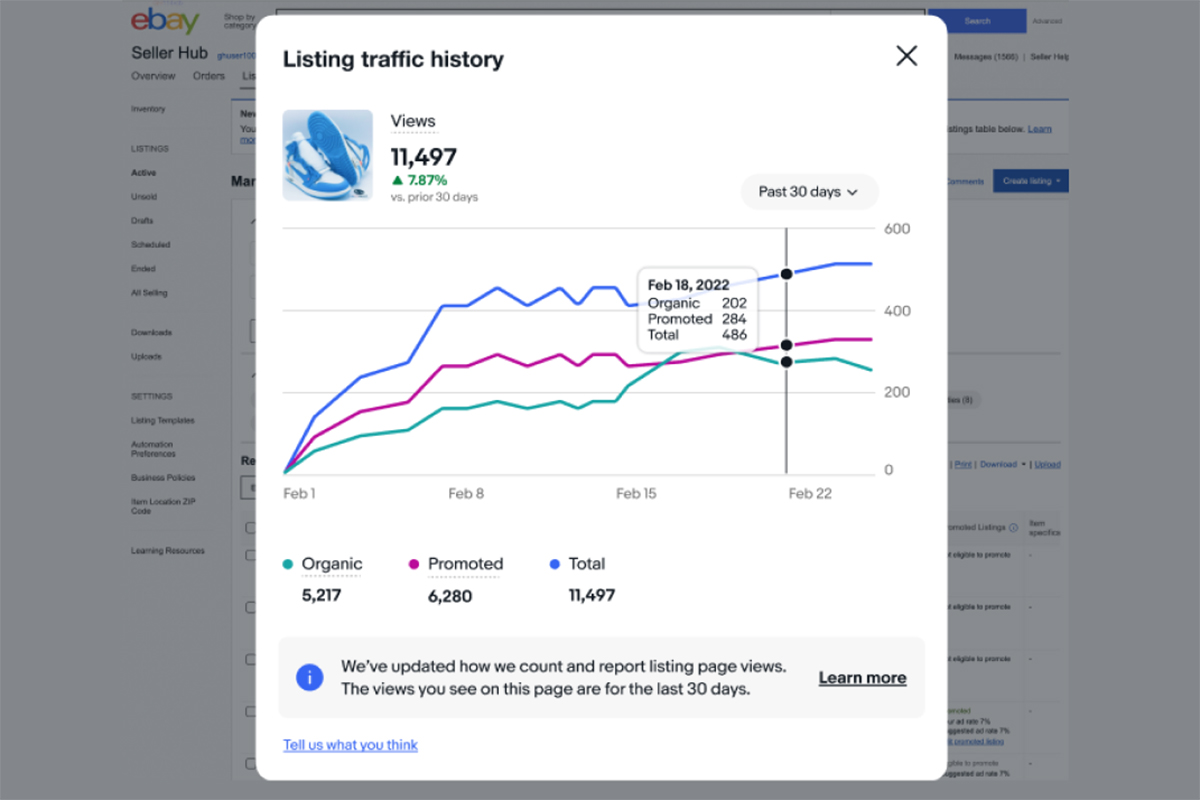The webpage from eBay displays a detailed listing traffic history for an item. At the top of the page, a title reads "Listing Traffic History," adjacent to a close (X) icon. An image of blue and white sneakers is prominently featured, accompanied by a statistic showing "Views: 11,497" with a green up arrow indicating a 7.87% increase in views compared to the previous 30 days.

Below this, a chart illustrates the traffic trends over the past 30 days, with three distinct lines representing different types of traffic: organic (green), promoted (purple), and total (blue). The total traffic, indicated by the blue line, consistently remains the highest. For example, on February 18th, 2022, the data shows 202 organic views, 284 promoted views, and a total of 486 views. The graph reveals a general upward trend, with occasional fluctuations where organic views momentarily surpass promoted views, though promoted views typically lead.

At the bottom of the page, a note informs users, "We've updated how we count and report listing page views. The views you see on this page are for the last 30 days." The page also features two buttons: a black "Learn More" button, and a blue "Tell Us What You Think" button. The majority of the webpage is set against a gray background, and the colorful eBay logo is visible, indicating the site's branding.